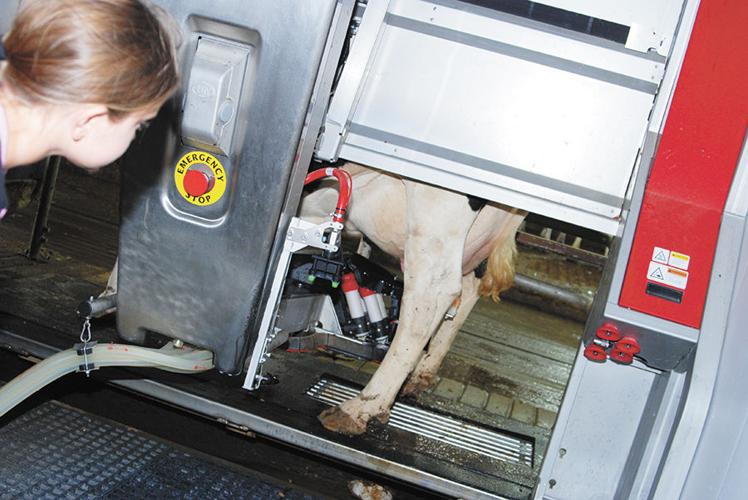The image depicts a metal milking machine stationed outdoors, featuring a black and white cow connected to milking pumps. The cow is positioned centrally within the machinery, which includes four white tubes attached to its udders, highlighting the milking process. On the left side of the frame, a young girl is curiously peeking down at the machine, examining the cow and its operation. Prominently in front of her is an emergency stop button encircled by a yellow label with black text reading "emergency stop." A red caution banner hangs on the right, and beneath the setup is a metal floor with grates. The details emphasize the industrial and functional aspects of this dairy apparatus.